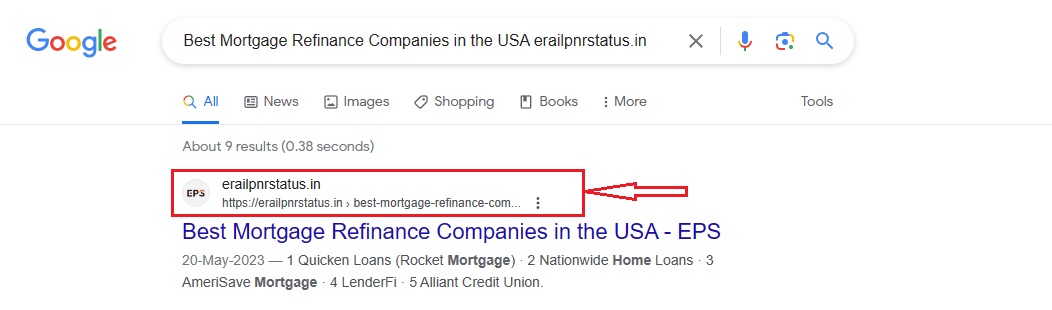This is a cropped screenshot of a Google search results page. In the top-left corner, the colorful Google logo is prominently displayed. To its right is the Google search bar, where the query "best mortgage refinance companies in the US in the USA eRail PNR status.in" has been entered. Below the search bar, the results are displayed, though it is indicated at the bottom of the page that approximately nine results were found, only one search result is visible. This solitary result directs users to the website eRail PNR status.in and is titled "best mortgage refinance companies in the USA."